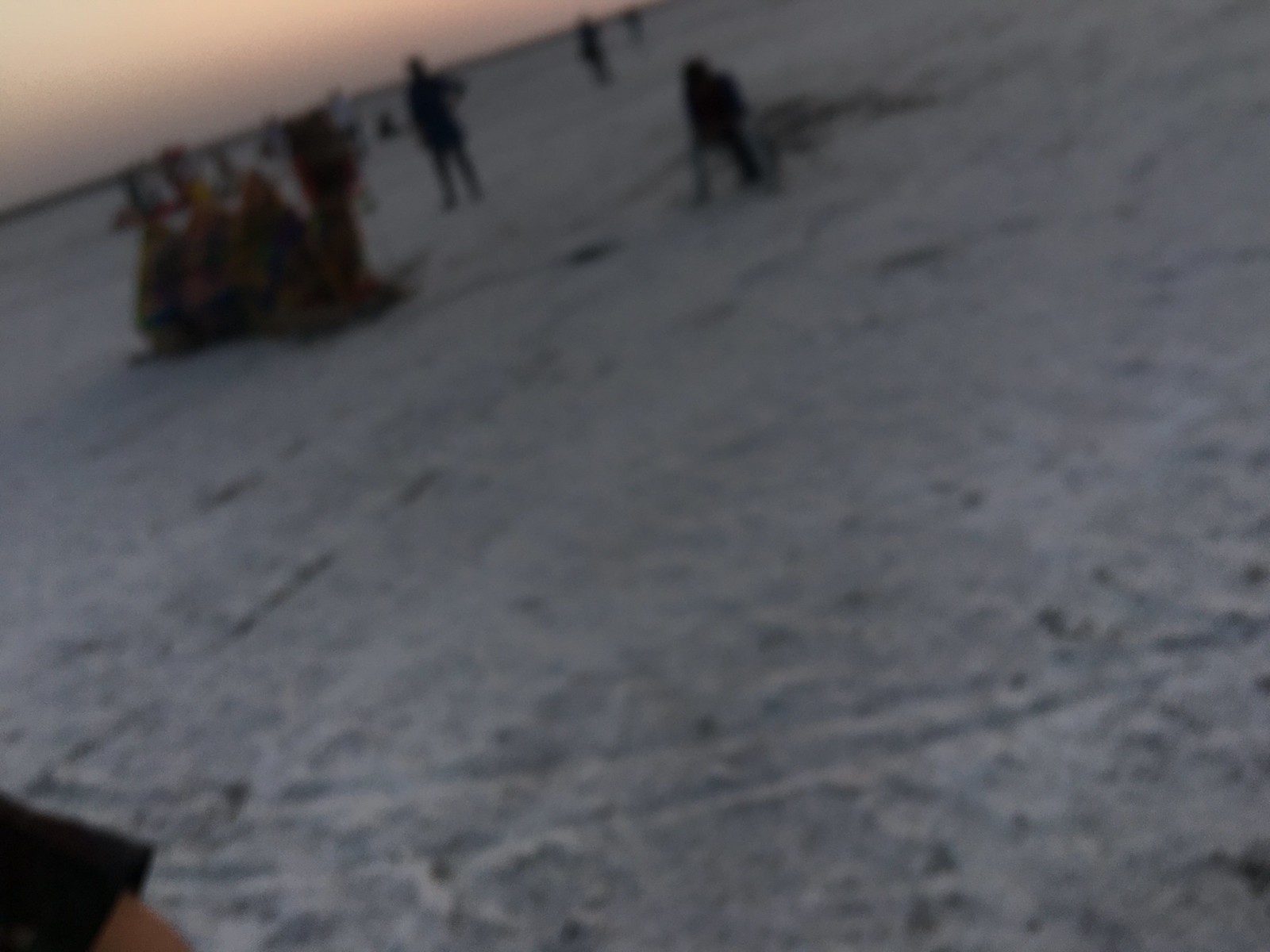The image depicts an outdoor setting during the evening, characterized by a brownish-white, desert-like landscape covered with snow. The top left corner features a large, three-humped camel with brown fur, sitting down with its arms tucked under its chest. Numerous people, dressed in winter clothing predominantly black, are scattered across the scene. A person's arm, clad in a black sleeve, intrudes into the bottom left corner of the image. The background shows a blurry field with some foggy or orange-hued sky elements, adding to the indistinct and hazy ambiance.